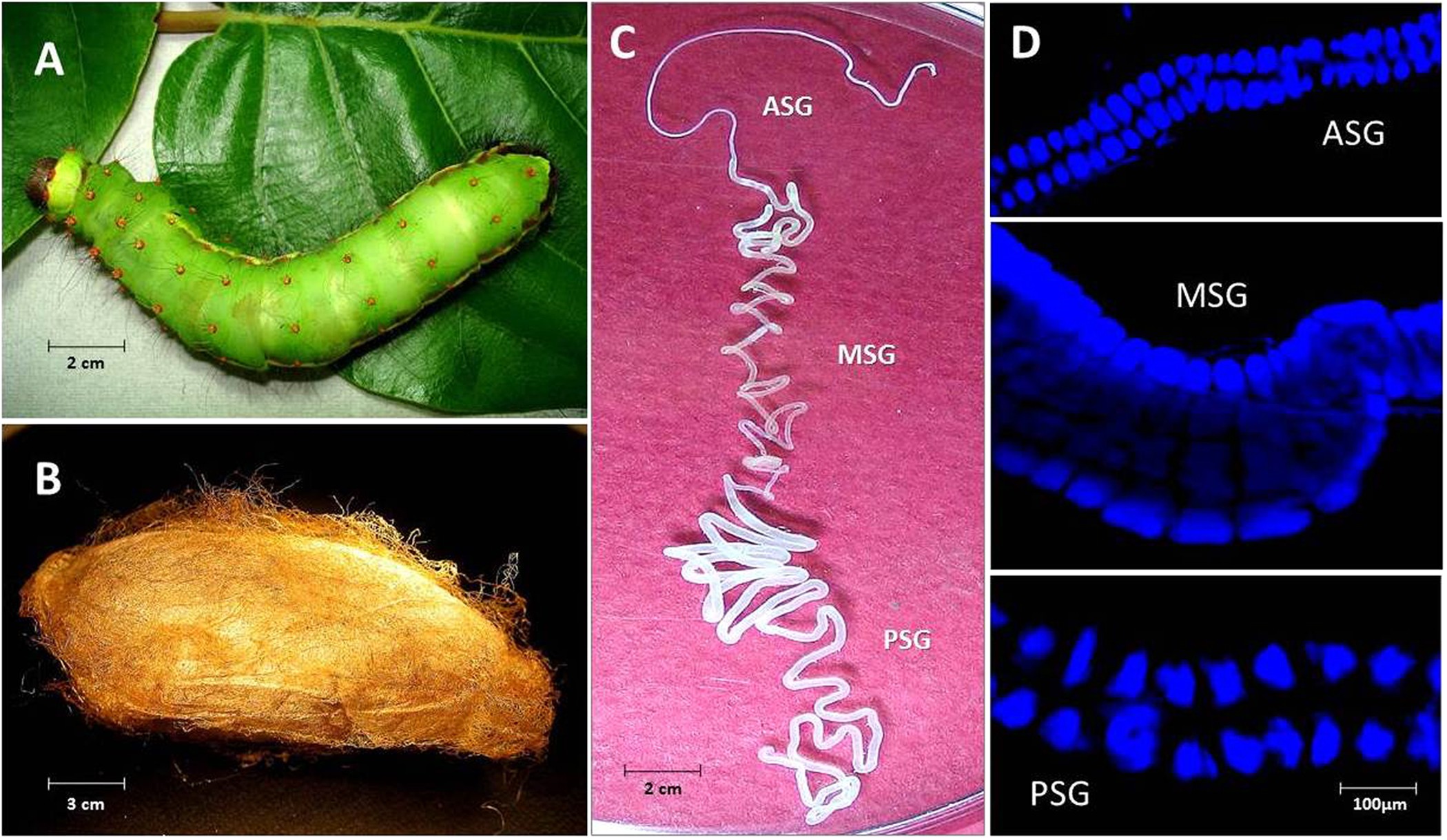The image displays a detailed collage segmented into four sections labeled A through D, each showcasing different stages and parts of what appears to be a caterpillar or silkworm. In section A, the top left, there is a close-up photograph of a plump green caterpillar resting on a leaf, accompanied by a two-centimeter scale for size reference. Below it, in section B, is an orange and yellow cocoon or similar construct set against a black background, also with a size guide. The central image, section C, presents a long, worm-like structure, segmented and labeled as ASG, MSG, and PSG, showing a continuum from thin to thicker segments, each part meticulously marked by a scale. On the right side, section D delves deeper with individual close-ups of ASG, MSG, and PSG, each depicted on a black background with intricate blue lines, possibly representing anatomical or internal features using what seems to be x-ray or chemical imaging techniques.